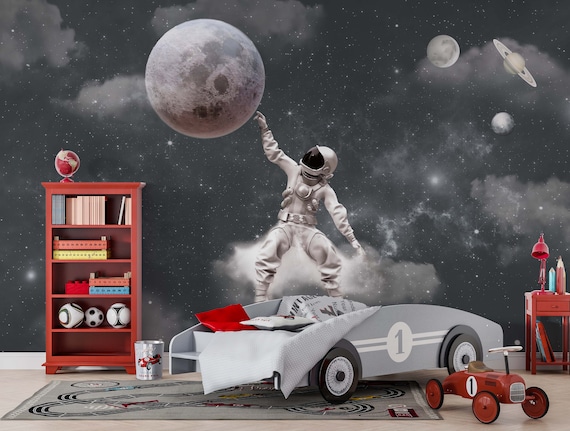The image appears to be a highly detailed and imaginative children's bedroom, possibly AI-generated or heavily photoshopped. The backdrop features a cosmic theme with a dark grey-to-black sky speckled with little stars and cosmic dust. In the upper right corner, there are several moons and planets, along with a large, prominent moon in the center left. An astronaut, dressed in a full spacesuit, stands in the middle of the scene, reaching out to touch the moon. To the left of the astronaut, there's a reddish-mahogany colored bookshelf filled with books, a globe, soccer balls, and various other toys. On the bottom right, a small toy pedal car in red color can be seen. Below the astronaut, a gray racecar bed with the number one on it is positioned prominently. The right side of the image depicts a desk. The overall color palette includes tones of orange, dark red, yellow, black, gray, and blue, creating a vivid and playful outer space-themed environment.